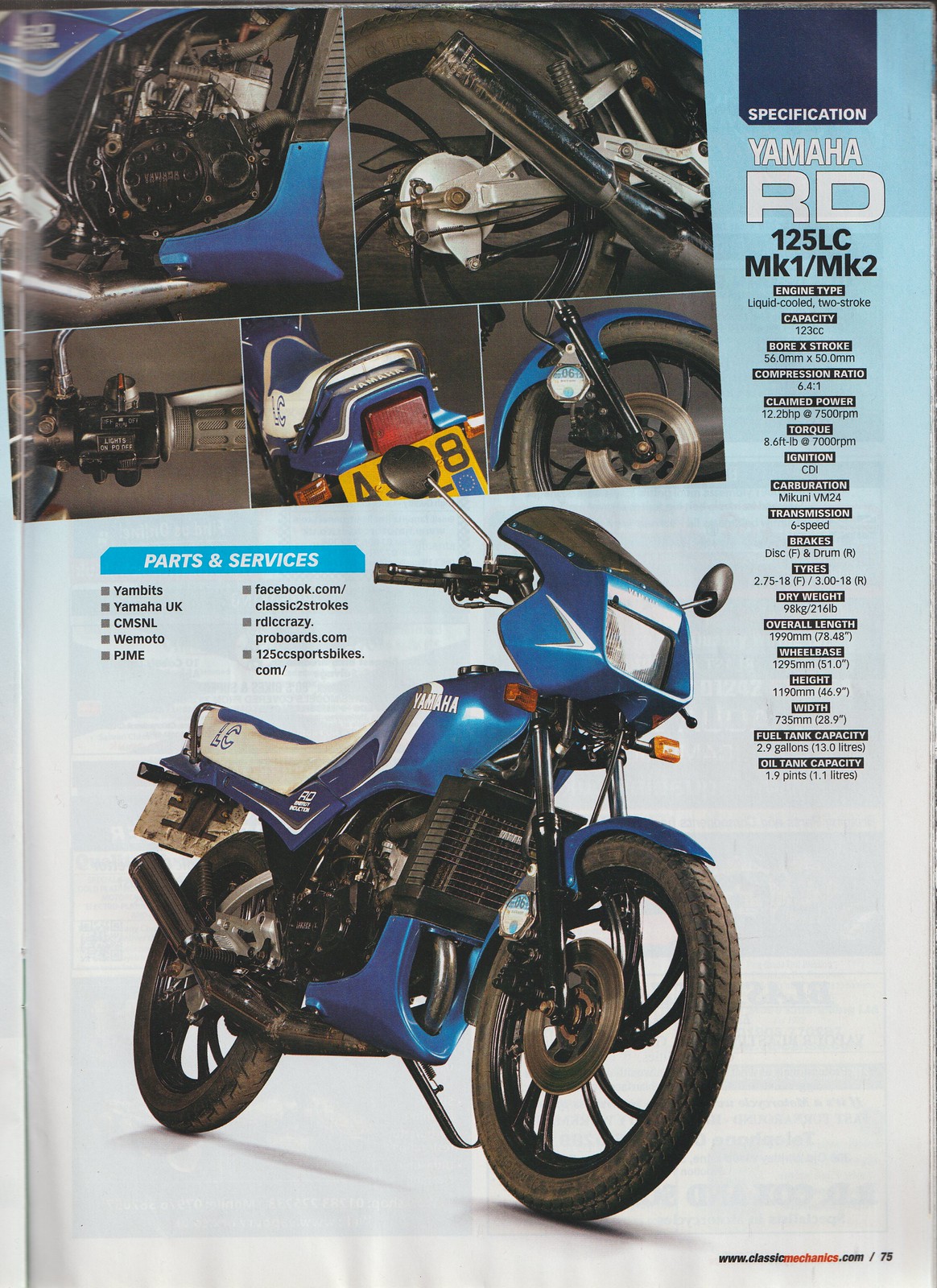This image is a tall rectangular page from a magazine or catalog, with a light blue background that fades to white at the bottom. It prominently features a Yamaha RD motorcycle ad, showcasing the bike's specifications and services. The main elements include a large illustration of a blue motorcycle with black and white accents, positioned towards the bottom half and tilted slightly forward to the right. Above this, in the top left corner, there is a collage of five close-up images highlighting various parts of the motorcycle. The top portion of the page contains bold white text that reads "Yamaha RD" on the right side, with additional small text that includes "125LCMK1-MK2." There is also a detailed list of parts and services displayed in white text over a blue rectangle located next to the top portion of the motorcycle. The yellow from the license plate adds a pop of contrasting color to the overall design. This detailed advertisement appears to be designed to both illustrate the motorcycle's features and provide potential buyers with service information.